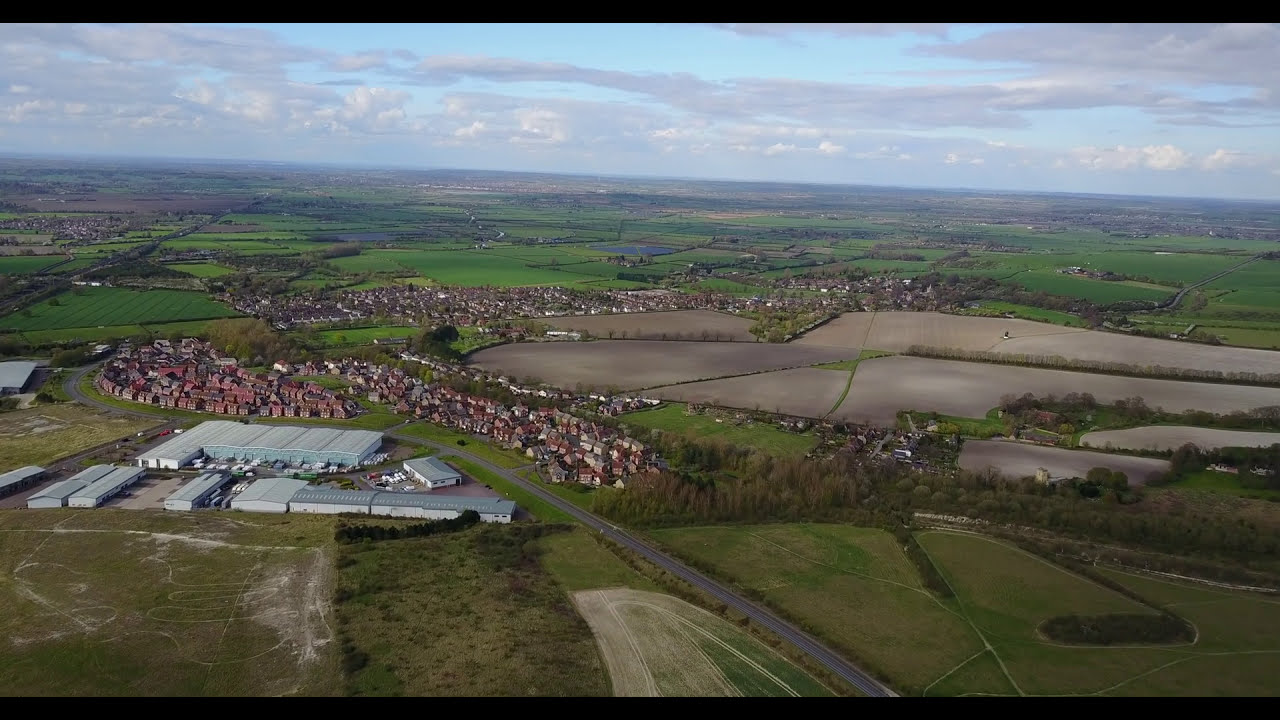This detailed aerial photograph, possibly taken from an aircraft or a high tower, captures a picturesque European village, likely situated in the Netherlands or Belgium. At the bottom left of the photo, there's a cluster of commercial or agricultural buildings, including white warehouses and a nursery, surrounded by white vehicles. These are adjacent to a narrow two-lane road that separates them from tightly packed, multi-storied residential houses. The homes, displaying a mix of historical European architectural styles, boast vibrant red roofs and various exterior colors predominantly in browns, beiges, reds, and pinks. 

Adjacent to the houses, large tilled fields with rich tan and brown soil stretch out, contrasting with lush green fields dotted with small grassy paths. In the right-hand side of the image, there are sections of empty paved areas with grassy dividers. Further in the background, more neighborhoods with similarly clustered homes and a couple of serene ponds are visible. The photo's fish-eye lens slightly distorts the horizon, but the scenic landscape of the countryside and its vibrant greenery remains clear, under a partly cloudy sky.